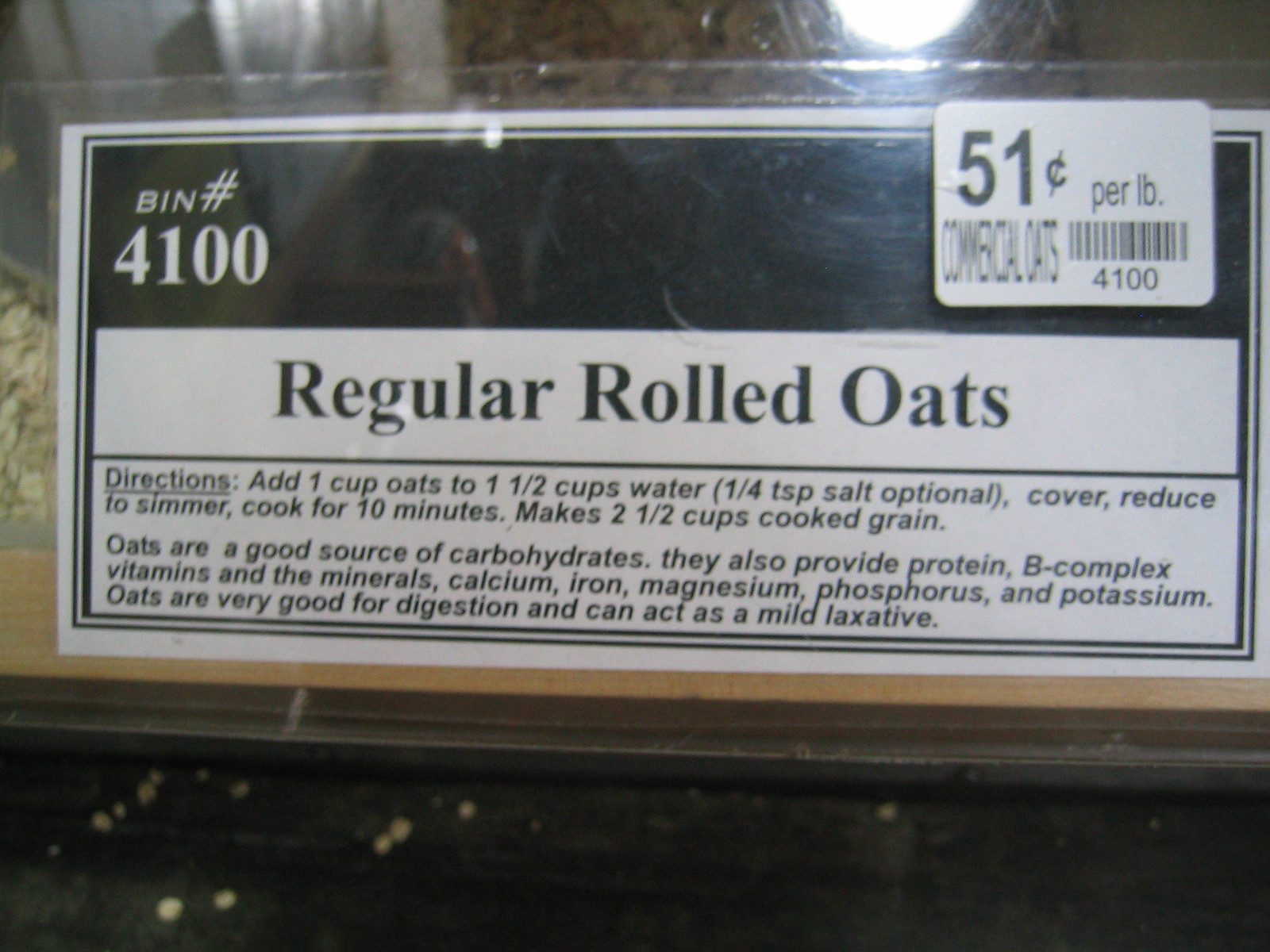This photograph captures a label from a bulk bin in a grocery store. The bins, made of clear plastic, are designed for scooping and purchasing bulk items. The label comprises two sections: the top section features a black bar with the text "Bin No. 4100," and the bottom section consists of a white bar with the text "Regular Rolled Oats." Detailed cooking instructions are provided: "Add 1 cup of oats to 1 1/2 cups of water (1/4 teaspoon salt optional). Cover, reduce to simmer, and cook for 10 minutes. Makes 2 1/2 cups cooked grain." Additionally, there is a sticker indicating the price, "$0.51 per pound," along with a barcode.